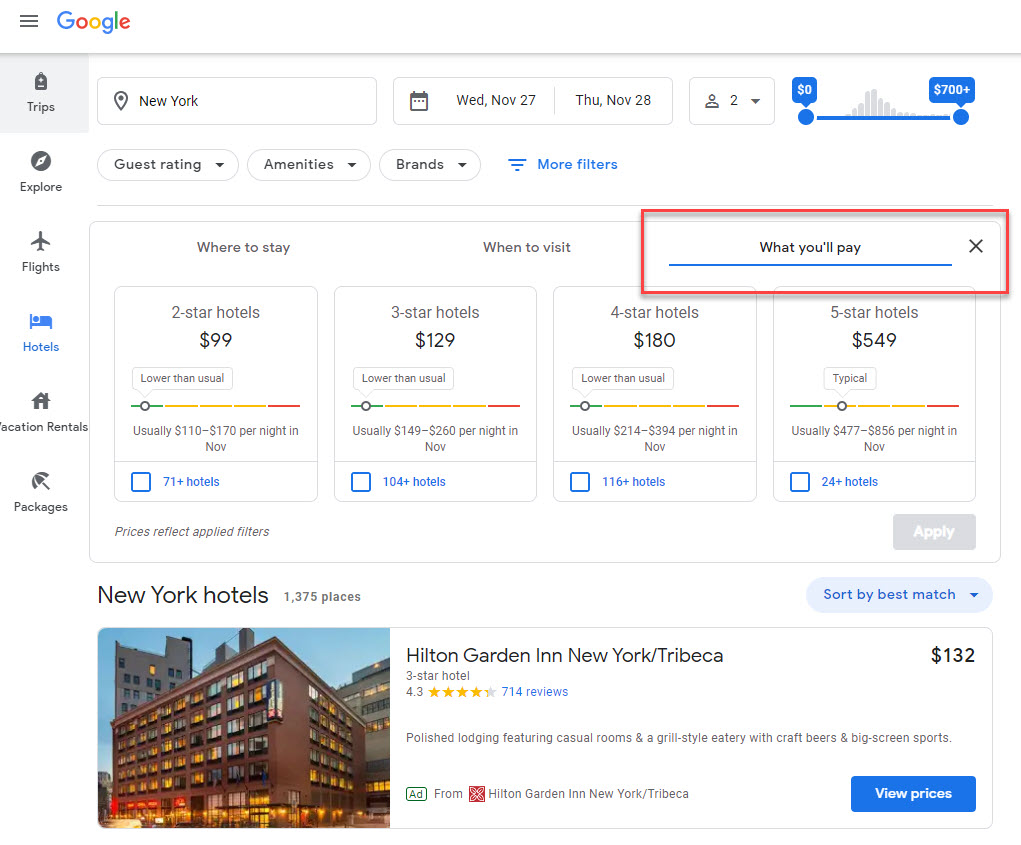This screenshot from Google Travel features a clean, white background. In the top left corner, the familiar Google logo stands out with its colorful letters: a blue "G," red "O," yellow "O," blue lowercase "g," green "l," and red "e." Below the logo is a thin line, followed by a sidebar menu on the left, listing options from top to bottom: "Trips," "Explore," "Flights," "Hotels," "Vacation Rentals," and "Packages." The "Hotels" option is highlighted in blue, indicating the current page.

At the top of the main section, the selected location is New York with check-in on Wednesday, November 27th, and check-out on Thursday, November 28th, for two guests. Below this, a highlighted section titled "Where to stay, when to visit, and what you'll pay" is framed by a red rectangle. This section allows users to filter hotel choices by star rating.

The categories are set up in rectangular boxes with price ranges and availability. Two-star hotels are listed at $99 per night, normally ranging from $110 to $190, with over 71 options available. Similarly formatted information is presented for three-star, four-star, and five-star hotels. The five-star hotel category shows a price of $549 per night.

Beneath these filters is a specific hotel listing for "Hilton Garden Inn New York/Tribeca," a three-star hotel with a Google rating of 4.3 out of 5 stars. The price for this listing is $132 per night. A photo of the hotel exterior is shown on the left, depicting a brick building approximately five stories tall, photographed during twilight.